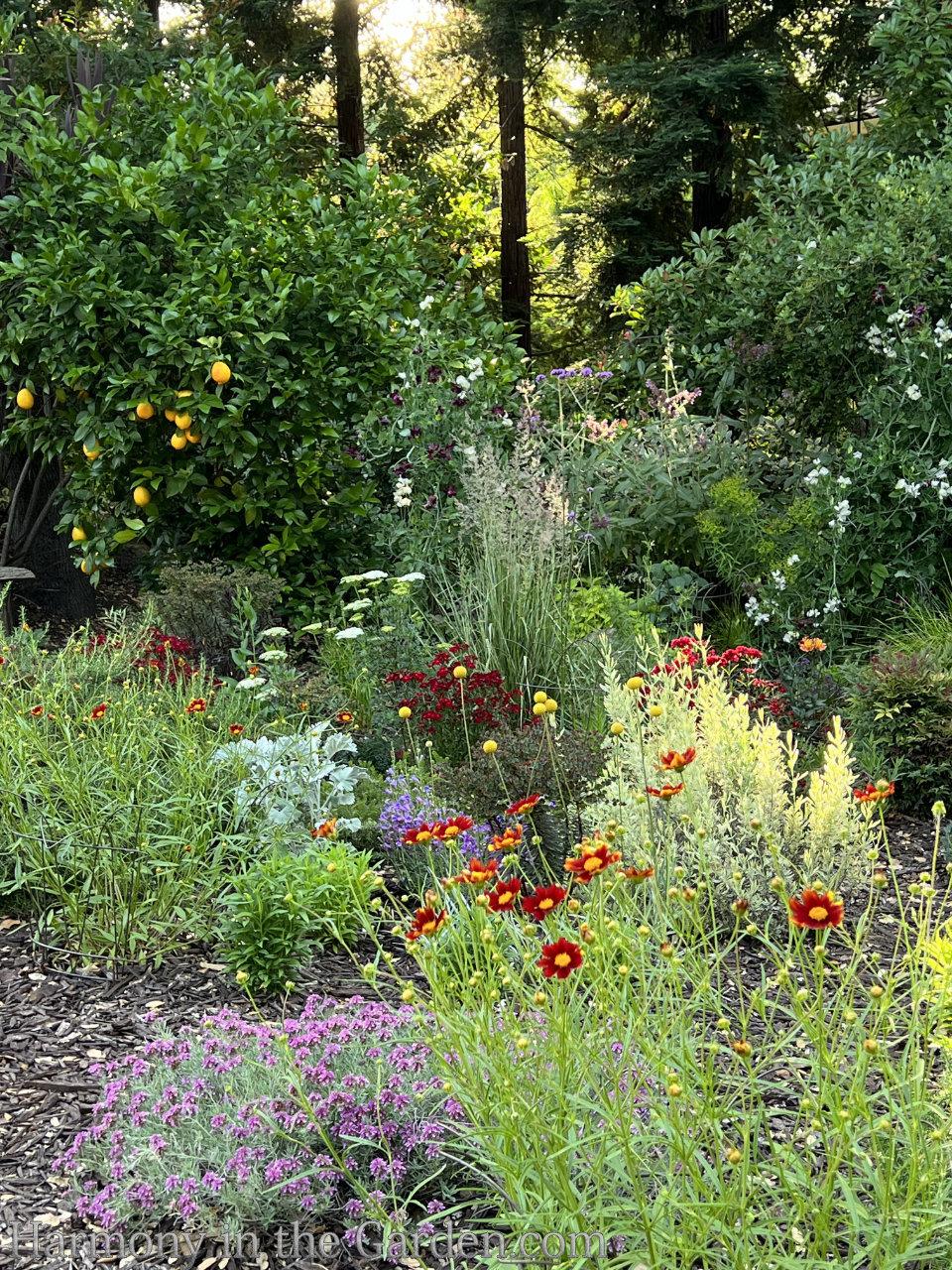This vibrant portrait-oriented photograph captures an outdoor flower garden rich with diverse and colorful vegetation, set against a serene woodland backdrop. The foreground is dominated by an array of wildflowers flourishing in mulched soil, with a few bare patches adding texture. Prominent among these are small red flowers with yellow centers and purple ground-hugging blossoms. Alongside, there's darker green foliage encrusted with intricate purple blooms and varieties of flowers featuring red petals with yellow centers.

The garden's midsection showcases more vibrant plants: a tall bush on the left flaunts bright green leaves and yellow flowers, while to the right, a slightly less vibrant bush sports white flowers. Interspersed among these are sage-green plants with purple-blue flowers, further diversified by additional bushes adorned with purple, red, and white flowers.

In the background, towering evergreen trees—likely pines—line the horizon with sunlight peeking through their branches. Closer in, smaller trees enhance the scene, with the leftmost bearing ornamental fruit, possibly kumquats or lemons. Overall, the garden, bursting with color and life, transitions seamlessly into the wooded backdrop, creating a harmonious blend of cultivated beauty and natural splendor.